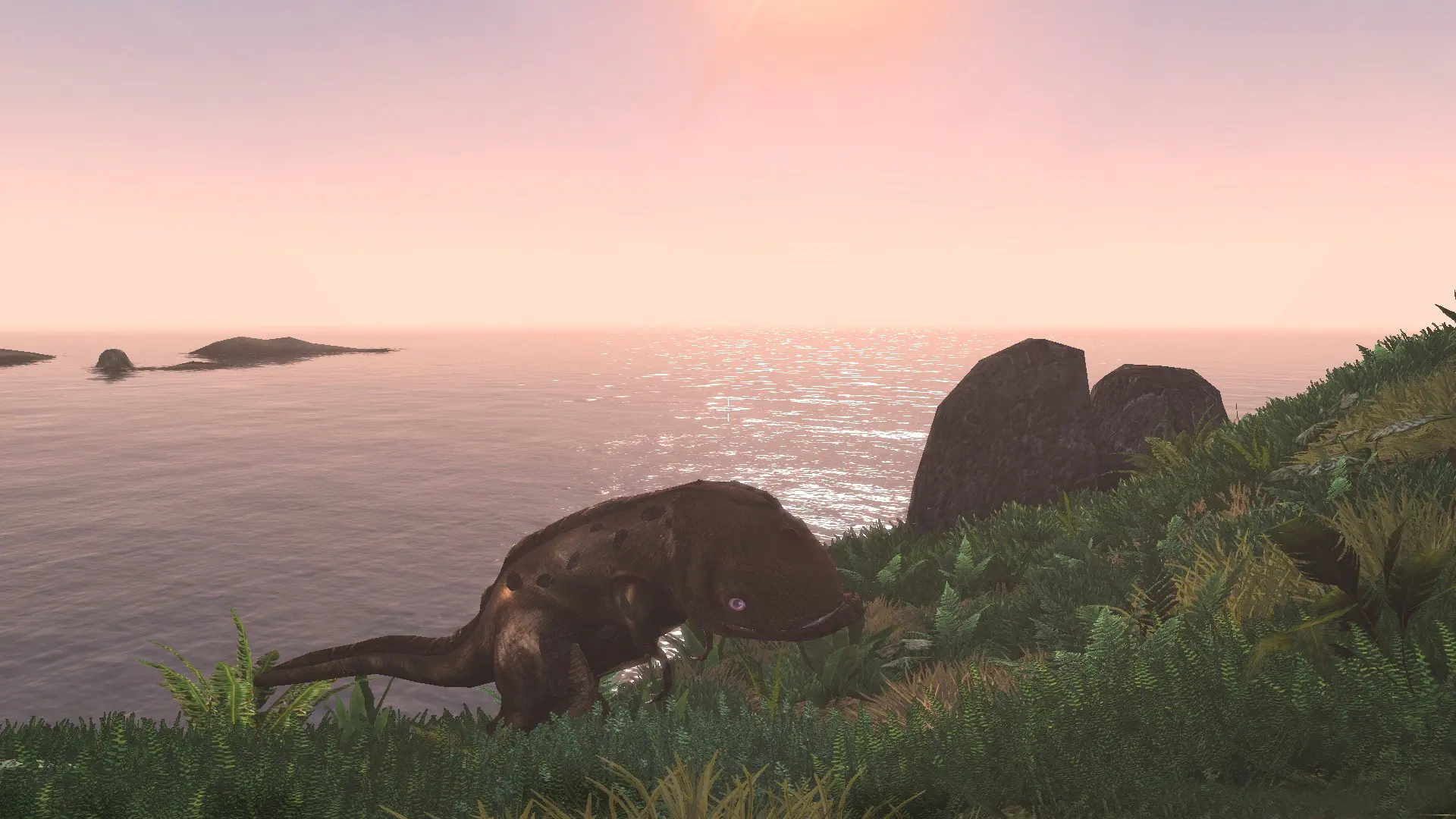The image depicts a vibrant, computer-generated fantasy landscape, likely from a video game. The scene features a pastel-colored sky transitioning from purples to pinks, with the Sun casting a pinkish haze at the top. Below, a serene ocean with gray-pink tinted water stretches out, dotted with a few rocks and possibly small islands. In the foreground, a hillside abundant with green grass and large leaves slopes gently towards the coastline. Amongst this greenery, a peculiar creature traverses the hill—resembling a cross between a fish and a small dinosaur, with thick back legs, a long tail, a wide, rounded face, and silver eyes. This fantasy creature stands out against the tranquil background, adding an element of intrigue to the serene, sunset-lit environment.